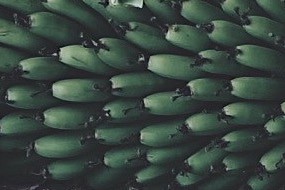This image appears to depict a close-up view of a large bunch of unripe bananas, although it has been rendered in an artistic style where the natural green colour of the bananas is represented in light blue. The bananas are tightly clustered together and oriented towards the left of the frame. Each banana has a distinct black tip, which is faithfully preserved in the stylized form. The background is a deep navy blue that enhances the contrast of the elongated, oval shapes of the bananas. There are some irregularities in the bananas' shapes and sizes, with about 30 bananas visible, each varied slightly in length with some ending in a touch of white. Additionally, a few white dots are scattered across the image, adding a decorative element to the composition.